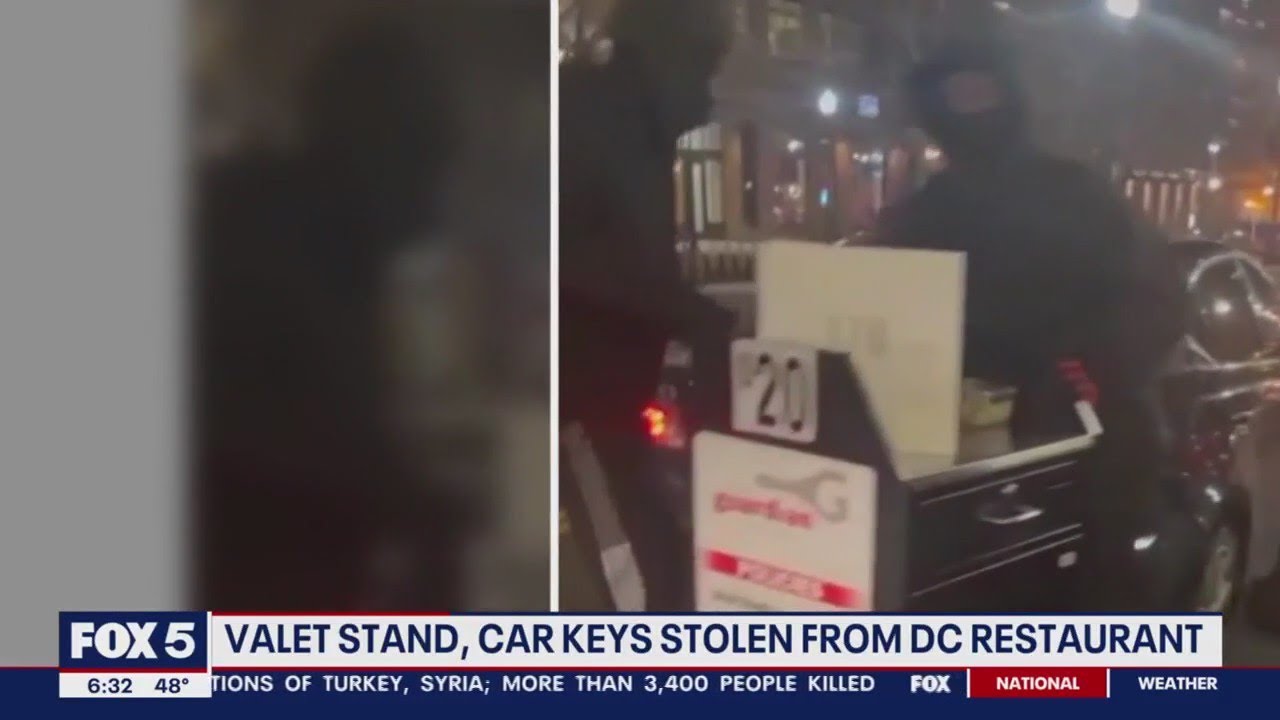The screenshot is from a Fox 5 news report captured at 6:32 p.m., with a temperature reading of 48 degrees. The primary headline announces "Valet Stand and Car Keys Stolen from a DC Restaurant," indicating a theft incident. Beneath this headline, a scrolling news ticker partially visible reads, "something of Turkey, Syria, more than 3,400 people killed," highlighting an international tragedy. The Fox 5 news logo and the word "National" are also present on the screen.

The image is divided into two segments. The left side is blurry and possibly viewed through a tinted window, making it difficult to discern details. However, it seems to show the shadowy outline of a person, presumed to be one of the robbers. The right side is clearer, displaying a building with a car parked in front, and two individuals who appear to be carrying furniture to the vehicle. The individuals are dressed in dark clothing, with one figure notably wearing a hood and covering the lower half of their face with a mask or bandana. The only visible skin is around their eyes. This chilling image seems to capture the moment the theft occurred, emphasizing the audacity of the crime.